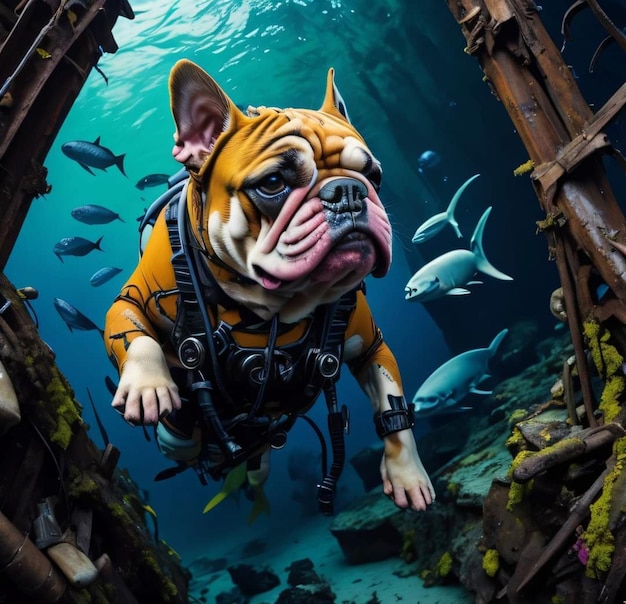This digital illustration, resembling AI-generated artwork, captures an underwater scene featuring a French Bulldog navigating the remnants of a shipwreck. The dog, a golden orange with white paws, a black nose, and pink jowls, is equipped with black scuba gear, including fins, a dive watch, and an oxygen tank, though he isn't using the tank or wearing a mask. He swims among blue-gray and darker blue fish without paying them any attention. The underwater environment is depicted with rusted metal beams and wooden planks from the shipwreck, white sand, and rocks on the ocean floor. Above, the ocean surface displays a teal hue with sunlit white highlights, adding to the scene's slightly surreal and digitally enhanced appearance.